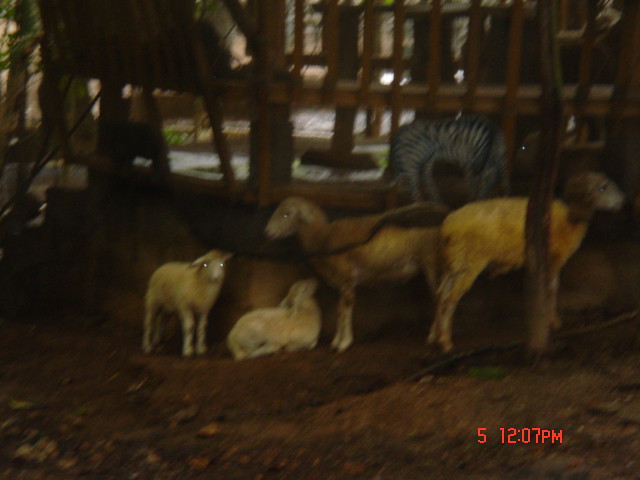This is an out-of-focus photograph capturing a group of trimmed sheep or possibly goats, standing on a dirt surface with wooden fencing in the background. The animals' fleece has been shorn, leaving them with bare coats. Most of the sheep are standing and gazing in various directions, with reflective eyes glinting from the camera flash. One sheep is lying on the ground in the center of the image, while to its left stands a smaller white sheep or lamb, and to the right, a larger sheep looks away. In the background to the right, partially visible behind the wooden fence or cage, there appears to be a zebra or a similarly patterned black and white animal, adding to the zoo-like setting of the scene. The timestamp "5, 12:07 p.m." is visible in the bottom right corner, suggesting the photo was taken sometime in the mid-2000s.